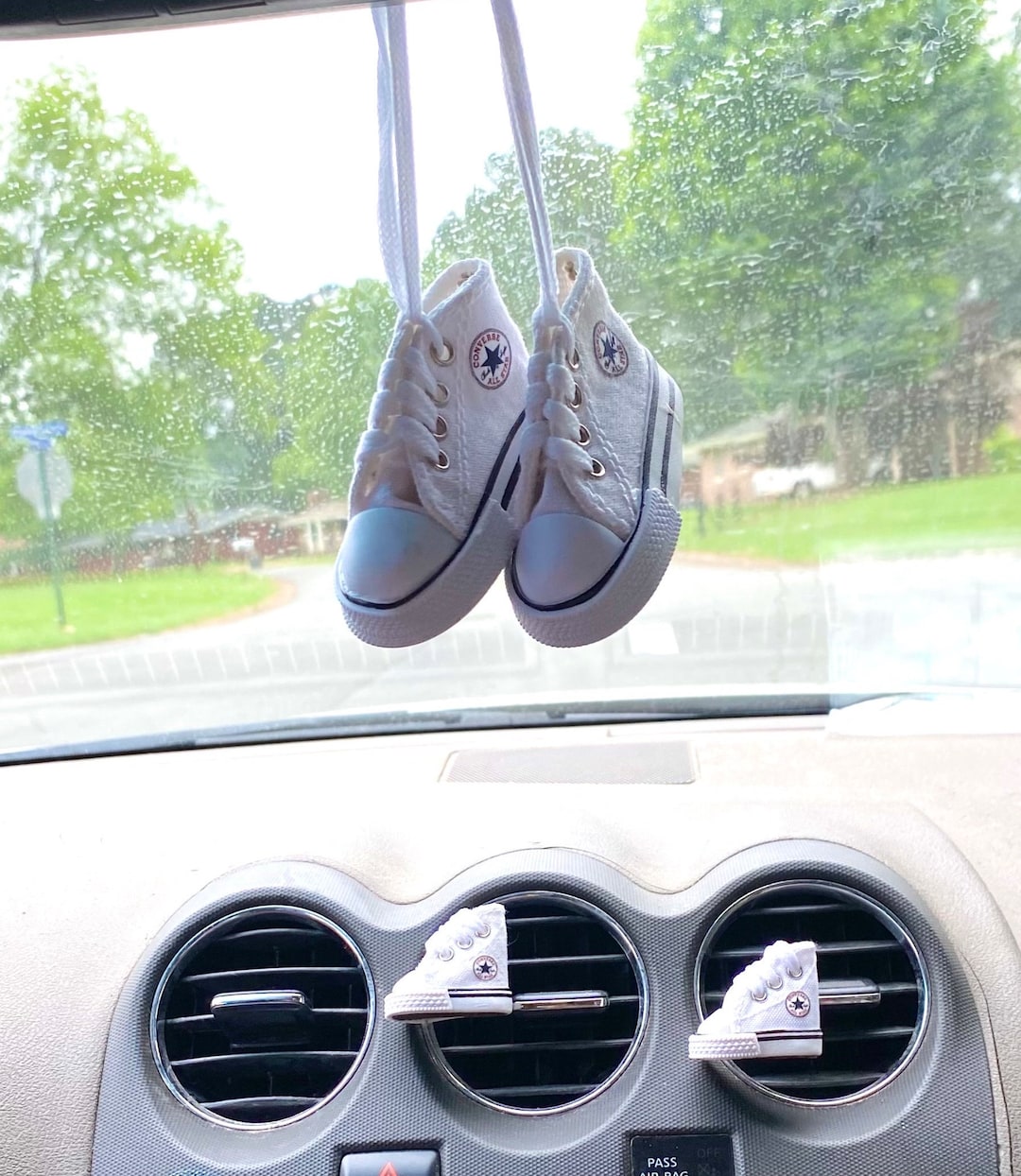The photograph captures an interior view from inside a car, looking out through the windshield. Prominently displayed is the car's dashboard, featuring three circular air vents. Attached to two of the vent levers are miniature sneakers, resembling white Converse, adding a quirky touch to the dash. Hanging from the rearview mirror, although not visible, are another pair of tiny shoes—cream and white baby sneakers, also mimicking Converse. Raindrops speckle the windshield, through which a bright, sunlit residential neighborhood can be seen. The road ahead is gray and wet, flanked by green trees and brick homes, creating a cozy, rain-washed streetscape.